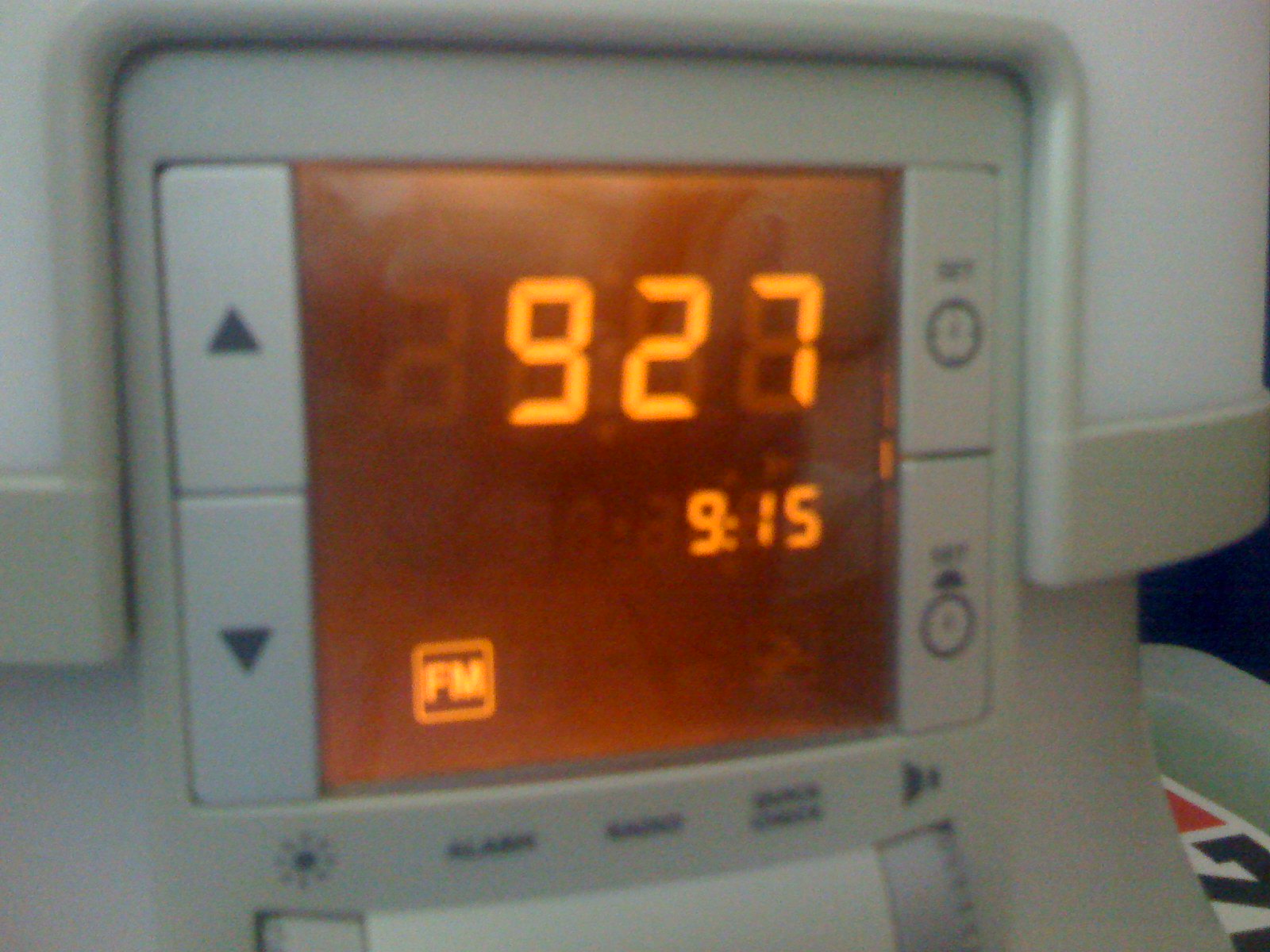The image showcases a close-up view of a white digital alarm clock. The clock features an orange-hued digital screen. Flanking the screen are buttons: on the left, there are two vertically-aligned buttons, one above the other, displaying up and down arrows. On the right side of the screen, there are two more vertically-aligned buttons, each marked with a clock symbol and a descriptive label, though the text is slightly blurred. Below the digital screen, there are several symbols and words: first, a star-shaped symbol, followed by the word "alarm." The subsequent text appears faint and possibly consists of two words stacked on top of each other. Lastly, there is a speaker symbol indicating audio functionality.